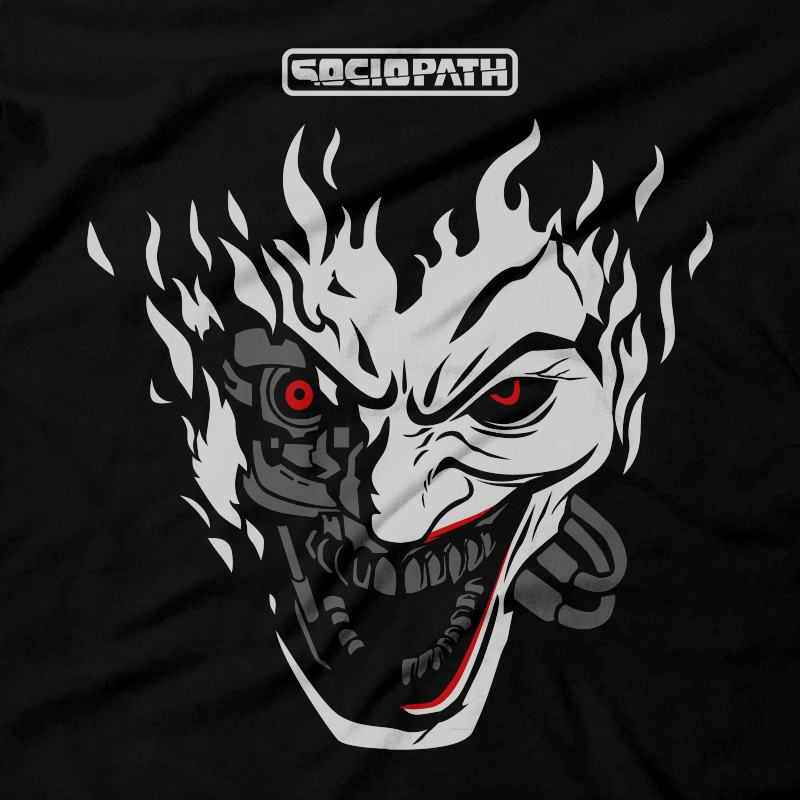The digital illustration features a hybrid face that combines elements of the Joker from Batman and a Terminator-like robotic structure. The face is split down the middle, with the right side depicting the Joker's light grey face with large, open, red-rimmed eyes, grey large teeth, and a red-lipsticked smile. The hair is stylized as white flames. On the left side, the face reveals a mechanical structure with steel skeletal features, grey in color, and connected by wires emerging from the neck into the jaw. The face is set against a wavy black fabric background, indicating it’s printed on a t-shirt. Above the Joker-Terminator face, there is a white rectangle containing the word "SOCIOPATH" in bold, thick, all-caps letters. The overall design evokes a sense of a villainous, demon-like character emphasizing the duality of organic and robotic elements.